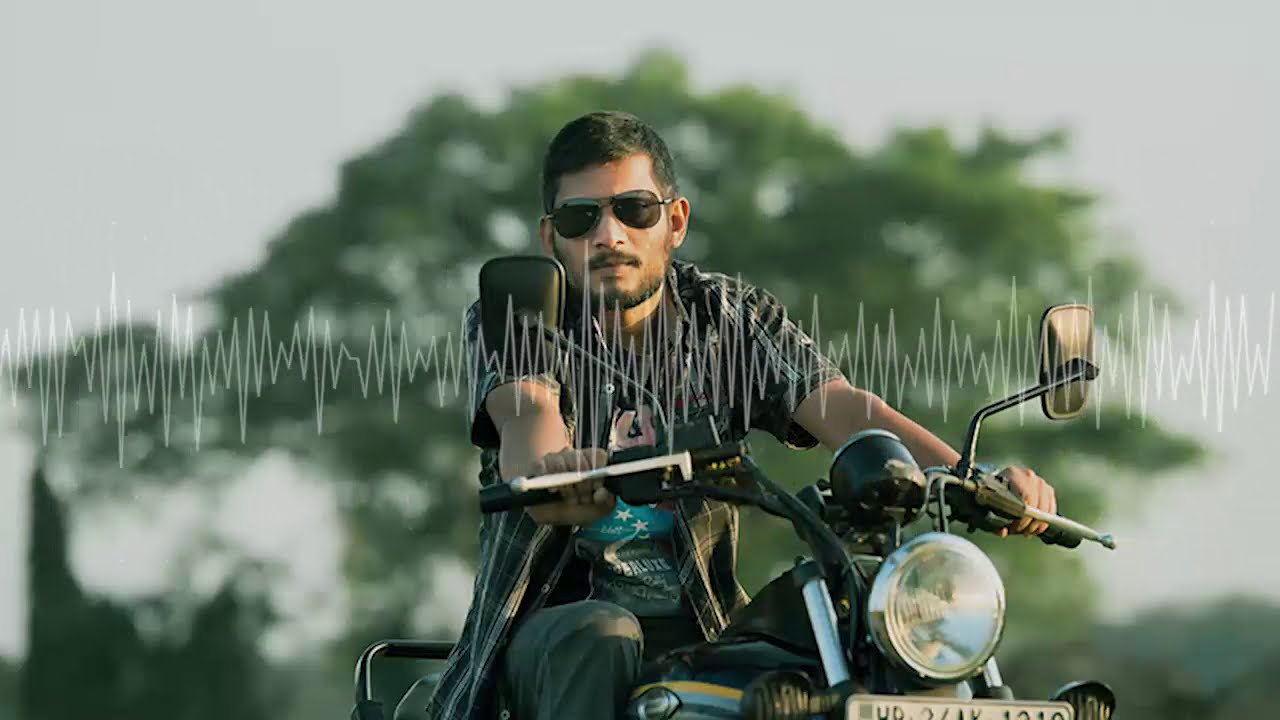This image captures a close-up of a young man, possibly Middle Eastern, sitting on a motorcycle that resembles a Harley Davidson. It's a bright day, evident from the large, blurred green tree in the background. The man is posing with his hands on the handlebars, looking directly at the camera. He sports dark sunglasses, short dark hair, a goatee, and a stubble beard. He is dressed in a black short-sleeved t-shirt featuring some sort of illustration, paired with black jeans. The motorcycle has a prominent front lamp and a speedometer behind it. Notably, there is a foreign license plate on the front, indicating the image was taken outside the United States. An unusual feature of this image is the white squiggly lines resembling a sine wave, running horizontally across the center from left to right.